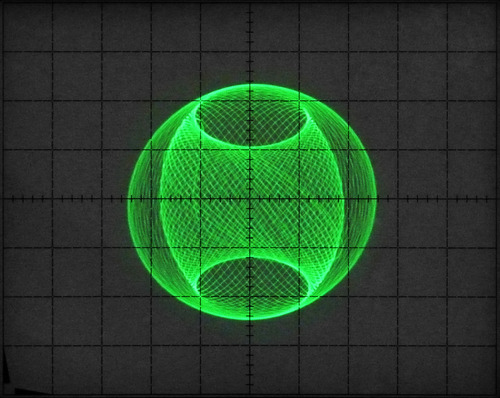The image depicts an abstract, computer-generated scene with a geometric composition. At the center of the image is a bright neon green sphere, intricately detailed with numerous fine lines that add a three-dimensional effect. Embedded within the sphere is an oval-shaped object with darker openings at the top and bottom, resembling a cylinder or possibly a tornado-like form. Surrounding this central sphere is a crosshair or target-like grid, consisting of black dotted lines that intersect in the middle, extending horizontally and vertically. The backdrop features an evenly spaced, gray square grid, creating a contrasting neutral background for the vibrant central elements. The overall style gives a sense of immersive depth and complexity, highlighting an intriguing blend of geometric shapes and abstract design.